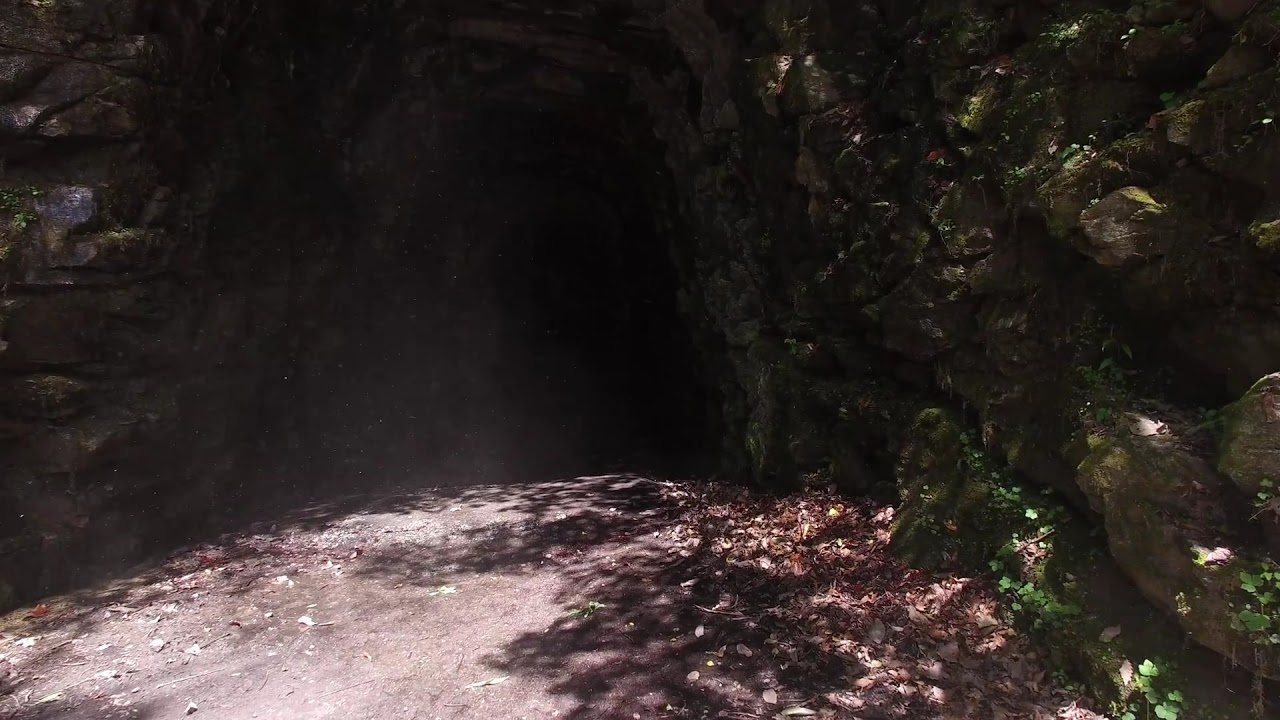This photograph, taken during a sunny day, captures the entrance of a mysterious cave nestled between tall cliff sides filled with rocks and ivy. The scene is viewed from ground level, with a hard-packed brown dirt path leading up to the cave. The sun shines brightly down from the top left, illuminating the ground in front of the cave and casting intricate shadows of ivy leaves to the right. The cave entrance, standing tall and narrow and estimated at about 30 feet high, creates a stark contrast between the illuminated exterior and the black, impenetrable darkness within. The left side of the cave entrance is somewhat obscured by the direction of the light, while the right side remains shrouded in deep shadow. Scattered dead leaves lie at the entrance, adding to the cave's enigmatic ambiance. The rough rocky walls on either side of the cave are adorned with dense foliage and vines, enhancing the natural and untamed allure of this secluded spot.